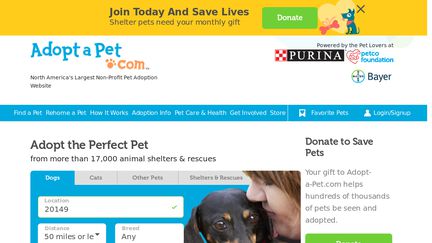This color screenshot showcases a web page from adoptapet.com, North America's largest non-profit pet adoption website. The website header features "Adopt a Pet" in turquoise lettering, with "Come" in orange, and a paw print replacing the dot. A prominent yellow banner at the top urges visitors to "Join today and save lives. Sheltered pets need your monthly gift," accompanied by a green "Donate" button and a cartoon of a blue dog holding a red bone.

Below the main logo, a line credits the pet lovers at Purina, Petco Foundation, and Bayer for powering the website. A thin blue navigation bar offers links to essential sections: Find a Pet, Rehome a Pet, How it Works, Adoption Info, Pet Care and Health, Get Involved, Store, Favorite Pets, and Login/Sign Up. The main focus area invites users to "Adopt the perfect pet from more than 17,000 animal shelters and rescues."

Highlighted search parameters include categories like Dogs, Cats, Other Pets, Shelters, and Rescues. The “Dogs” section is currently selected, with search filters set to a location of 20149, a distance of 50 miles or less, and breed listed as "Any." 

The page also features a touching photograph of a woman looking down in profile towards the left, gently holding a small black and brown dog resembling a dachshund. To the right of the image, a call-to-action reads: "Donate to Save Pets. Your gift to adoptapet.com helps hundreds of thousands of pets be seen and adopted."